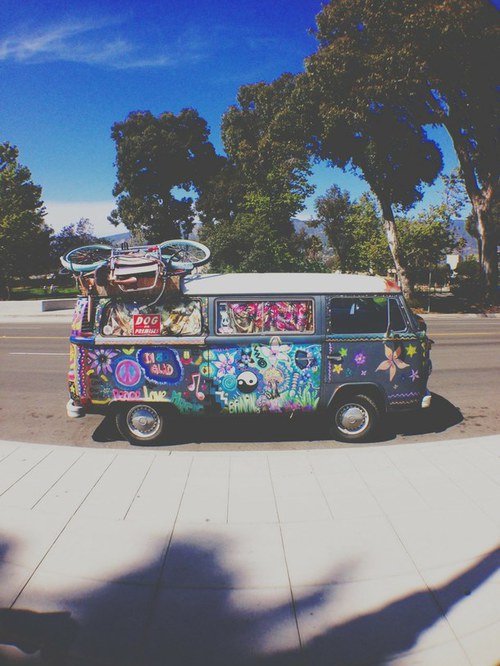The photograph captures a vibrant, decorated VW bus, emblematic of the 70s hippie culture, parked on a multi-lane street beside a sidewalk with square-shaped stone tiles. The right side of the bus is visible, adorned with an array of trippy and colorful designs, including peace symbols, Tao symbols, and a profusion of flowers in shades of white, black, blue, pink, green, purple, and more. Stars are also part of the artistic mix. Atop the VW bus, a bicycle and some luggage are strapped, accentuating its adventurous spirit. The backdrop features tall trees with green leaves, while the sky overhead is a beautiful blue with feathery white clouds, particularly prominent in the upper left-hand corner of the image.